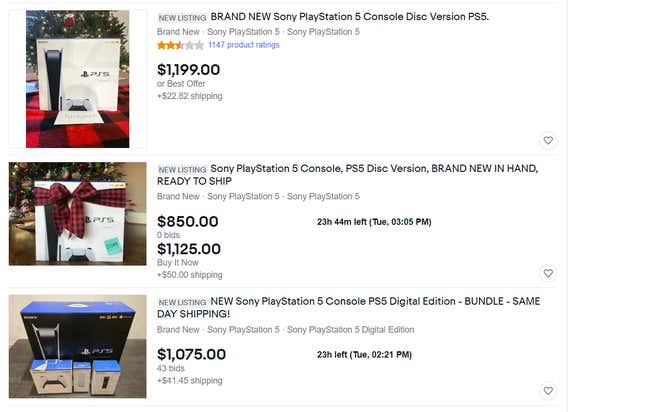**Detailed Product Listings for Sale**

**Product 1:**

- **Product Image:** On the left.
- **Product Name:** Brand New Sony PlayStation 5 Console Disc Version (PS5)
- **Additional Details:** Listed as a new product in gray text, with a repeat in black text: "Brand New Sony PlayStation 5 Sony PlayStation 5."
- **Rating:** 2.5 stars indicated by gray stars, with "1147 product ratings" in blue text.
- **Price:** $1,199 or best offer.
- **Shipping:** $2,282.

**Product 2:**

- **Product Image:** On the left.
- **Product Name:** Brand New Sony PlayStation 5 Console PS5 Disc Version
- **Additional Details:** Captioned as "BRAND NEW IN HAND READY TO SHIP" in capital letters.
- **Price:** $850 with zero bids, or $1,125 for the "Buy It Now" option.
- **Shipping:** Unspecified.

**Product 3:**

- **Product Image:** On the left.
- **Product Name:** New Sony PlayStation 5 Console PS5 Digital Edition
- **Additional Details:** Labeled as "BUNDLE SAME DAY SHIPPING!" in capital letters.
- **Price:** $1,075 with 43 bids.
- **Shipping:** $4,145.